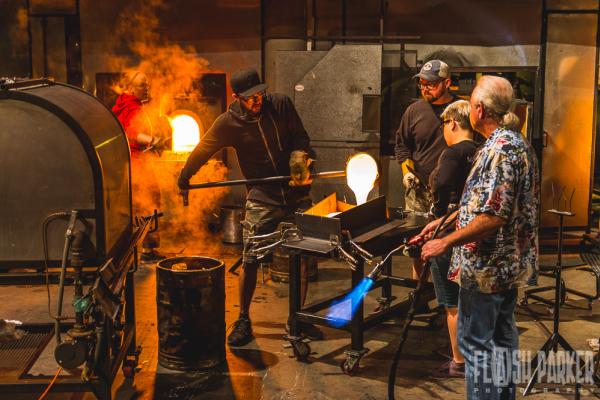The image depicts a scene in a bustling blacksmith shop or boiler room featuring four men immersed in different tasks. Central to the picture, one man in a black hat and gloves is carefully holding a long rod over a metal tray, from which a glowing ball of hot liquid metal drips steadily into the mold below. To his immediate right, a man wearing a ball cap and dark shirt stands attentively, observing this delicate operation. A third man, positioned slightly to the right and facing away, is donned in a dark top and blue shorts. Further in the background, close to a wall lined with pipes and what might be an incinerator or furnace, is a figure in an orange suit, enveloped in slight smoke as they maneuver beside the hot oven.

Adding to the scene's complexity, a fourth individual on the far right, with grayish hair tied in a bun and dressed in a multicolored shirt and jeans, holds a torch emitting a blue flame, contributing to the intense, fiery activities. Scattered around the workshop are various tools: a bucket, a drum, and a covered object with pipes and hoses that resembles a smoker. On the floor, a trash can is visible to the left of the man with the rod, and in the bottom right corner of the image, faint white text reads "Flash Parker," followed by an inscrutable line. The collaborative efforts of these skilled artisans highlight the traditional and intense nature of metalwork in this cramped, high-temperature environment.